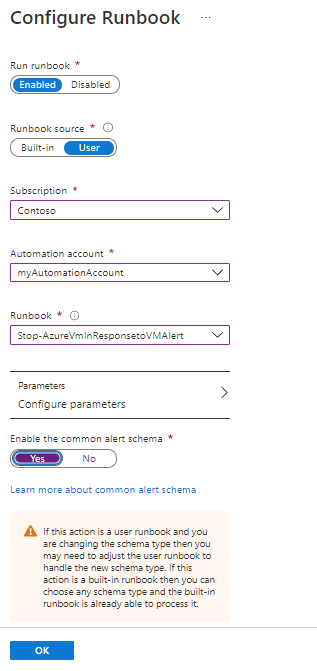The image depicts the configuration interface for a Runbook. At the top of the interface, the title "Configure Runbook" is displayed in bold black text. Below this title, a toggle option for "Run Runbook Enabled" is highlighted in blue, with the alternative option "Disable" adjacent to it.

Further down, there is a section labeled "Runbook Source," featuring two options: "Built-in" and "User." The "Built-in" option is highlighted in blue. Directly below this section, there is another labeled "Subscription," showing the selected subscription named "Contoso."

Proceeding further down, the "Automation Account" section lists "My Automation Account" as the selected account. In the "Runbook" section, a clickable link is provided for detailed Runbook information. 

Next, the "Parameters" section is labeled as "Configure Parameters." Below this is an option to "Enable the Common Alert Schema," with a choice between "Yes" and "No." The "Yes" option is highlighted in purple, located on the left side.

Following this, a light blue link reading "Learn More About Common Alert Schema" is provided. Below this link, a paragraph in small black text explains: "If this action is a user runbook, and you are changing the schema type, then you may need to adjust the user runbook to handle the new schema type. If this action is a built-in runbook, then you can choose any schema type, and the built-in runbook is already able to process it."

At the very bottom left of the interface, a blue "OK" button is positioned, with the word "OK" in white letters at its center.